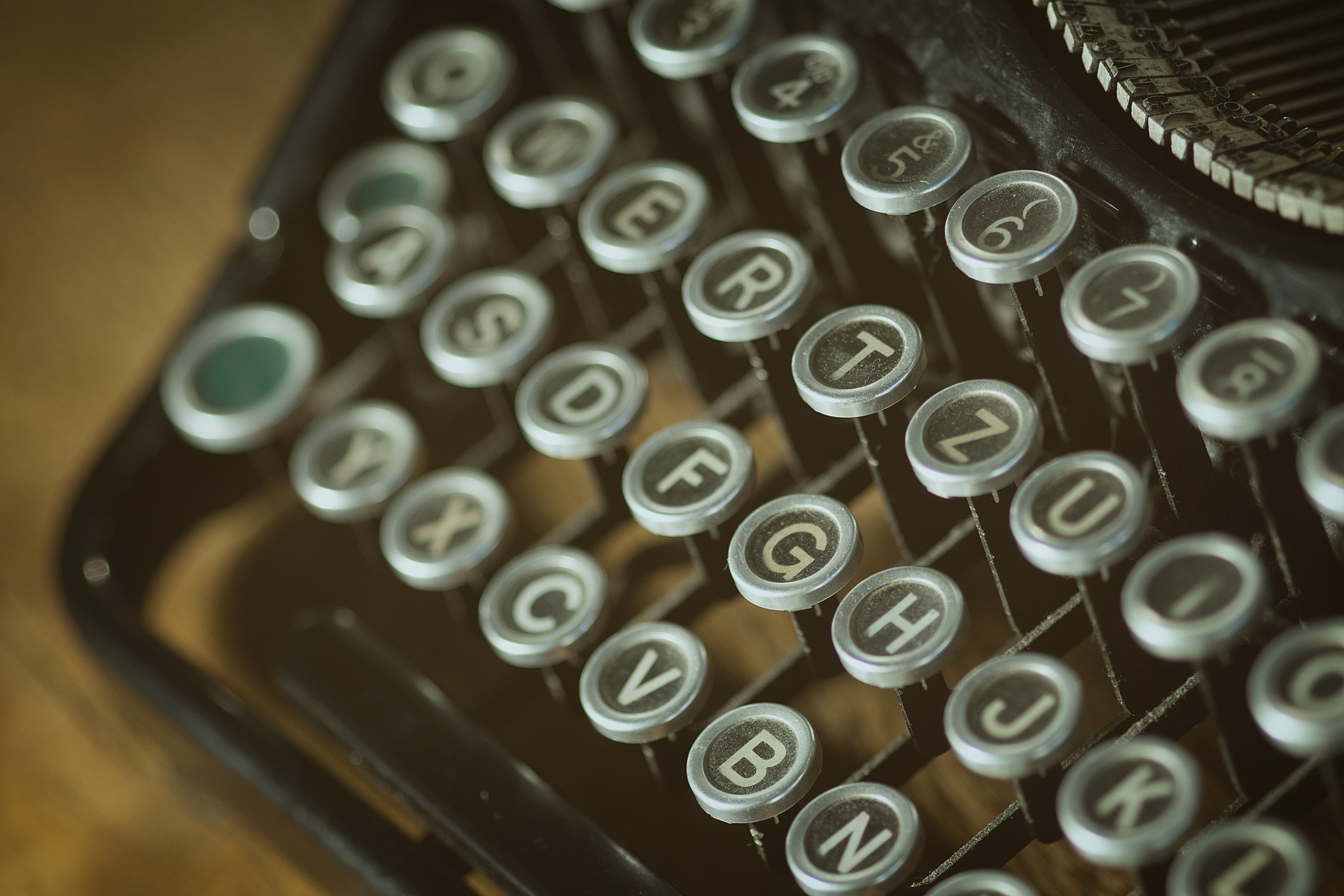This indoor color photograph presents a detailed close-up of an old-style manual typewriter, likely from the late 1800s or early 1900s. It captures a partial view of the typewriter, angled such that the back is cut off towards the top right, focusing instead on the array of round, silver-bordered keys which feature a black center with white letters. The camera primarily centers on the dusty keys, highlighting the prominent wear of time.

The keys are arranged in the standard QWERTY layout that we use today. On the top row, numbers 3 through 8 are visible. The second row reveals the letters Q, W (both slightly blurred), E, R, T, Z, U, with I and O blurred. The third row showcases a mix of blurred and clear keys: A and S (slightly blurred), followed by D, F, G, H, J, K (slightly blurred), and L (very blurred). The bottom row includes a larger green button, partially blurred Y and X, with clearer keys C, V, B, and N. Two distinctive green buttons stand out, one on the third row and a larger one on the bottom row, enhancing the nostalgic aesthetic.

In the background, the typewriter rests on a round desk, though the details around the typewriter remain blurry as the image singularly focuses on the keys. Slight hints of the manual key levers can be discerned, suggesting the mechanical process of the typebar striking the ribbon to imprint characters onto paper.